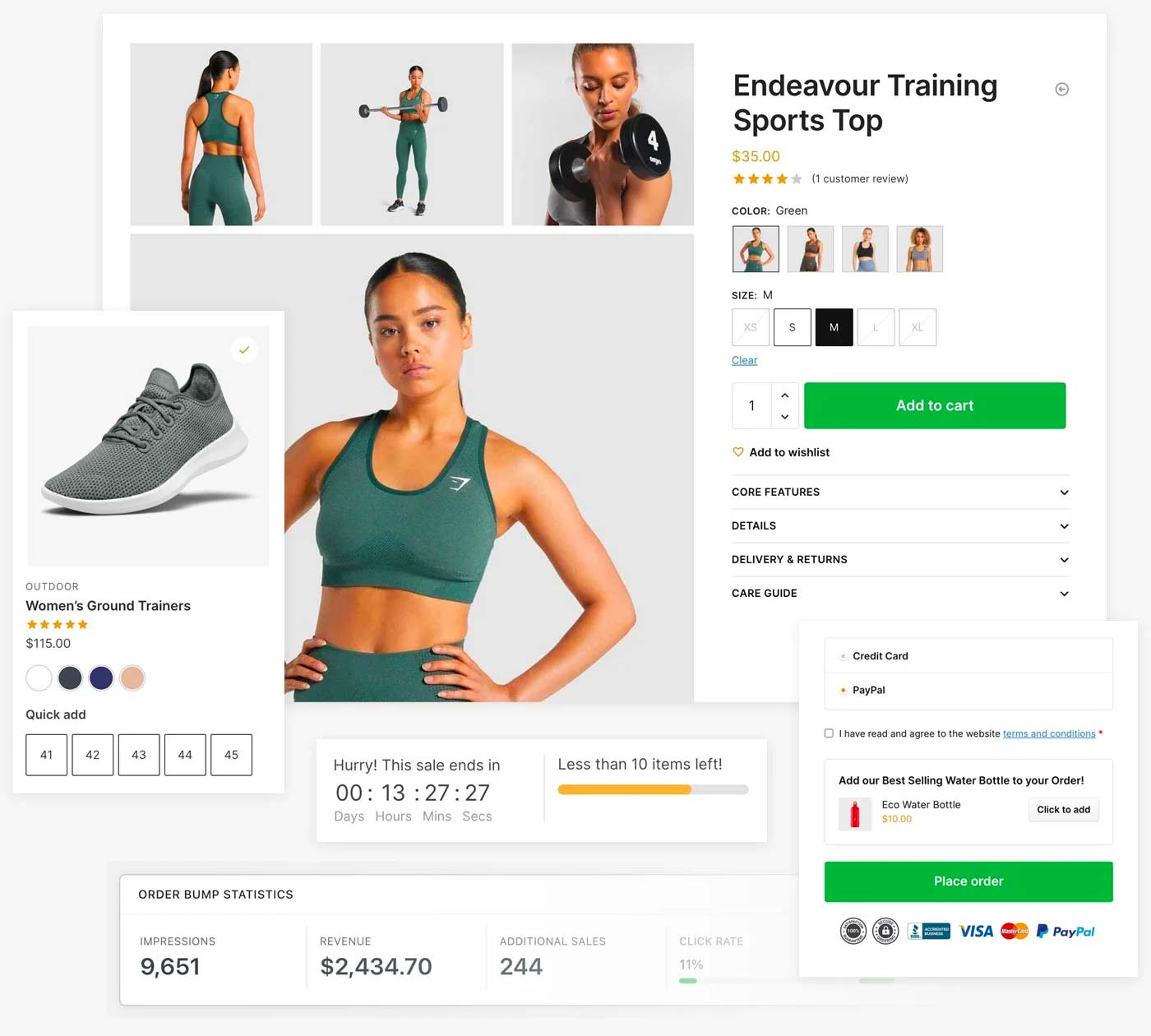The image depicts a web application interface showcasing a product page for a sports outfit. The background is white, highlighting various visual elements framed by the software window. Dominating the screen are multiple images of a woman dressed in a coordinated green sports tank top and green tights, paired with grey shoes that have white soles.

The main visual is a large photograph at the center, capturing the woman standing confidently with her hands on her hips. In the lower left corner of this photograph, the grey shoe with its distinctive white sole is visible. 

On the right side of the interface, there is a section dedicated to product information and purchasing options. At the top of this section, the text "Endeavor Training Sports Top" is prominently displayed in black. Beneath this title, there are selection options for choosing the size of the sports top. The option for size M is clearly highlighted within a black square, indicating it is the currently selected size. Towards the bottom of this section, there is a green "Add to Cart" button, inviting users to proceed with their purchase.